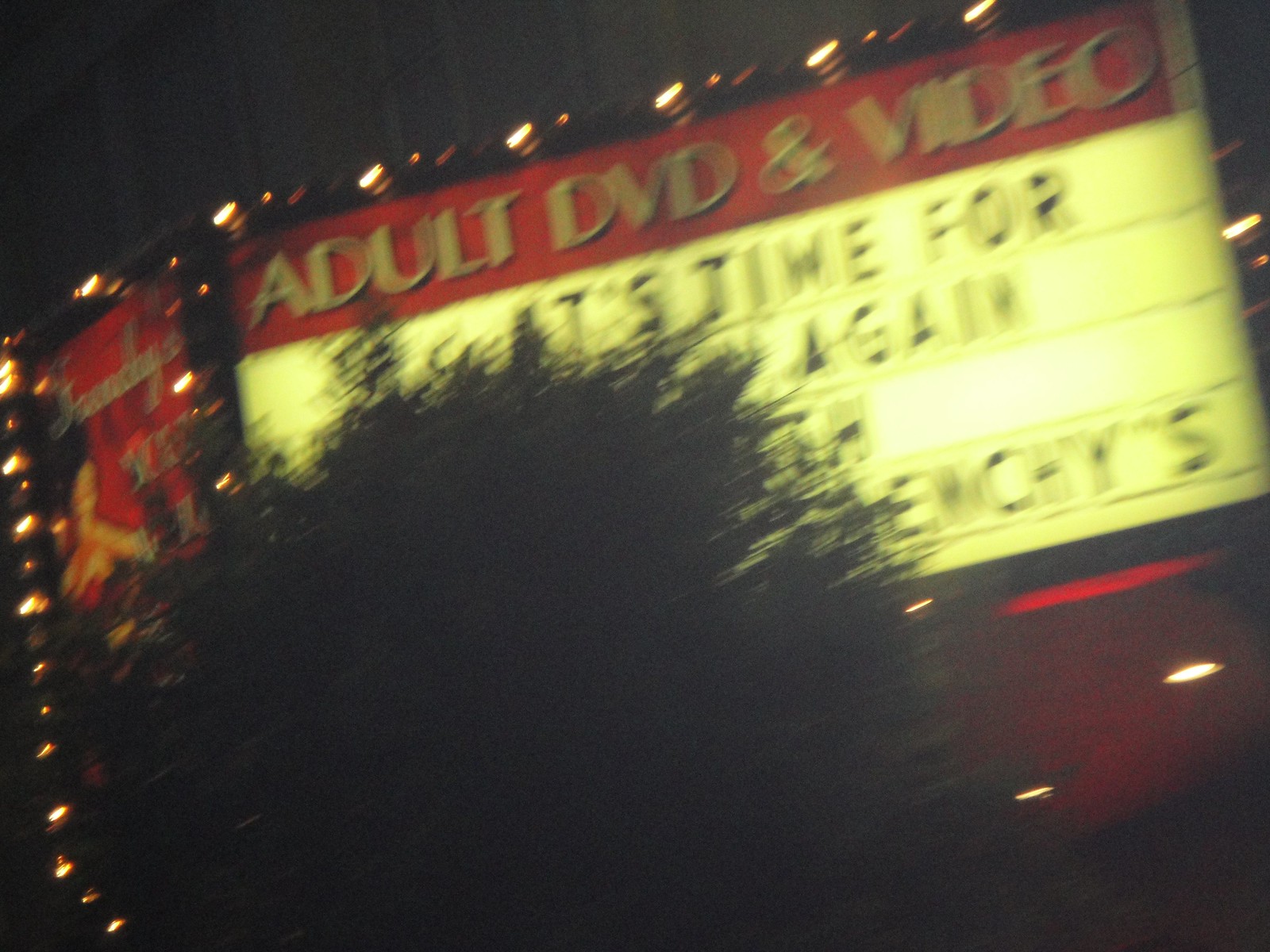A blurry and grainy freeze frame from a video filmed outside a large cinema, likely located in America or Canada. The brightly lit marquee, though distorted, prominently displays "Adult DVD and Video." Below this, the title of a film reads "It's Time For," but the remainder is obstructed by a large tree or bush. Despite the challenging clarity, some details of the cinema's chain of lights can be faintly discerned through the haze, resembling the view of an individual with astigmatism or a similar visual impediment.